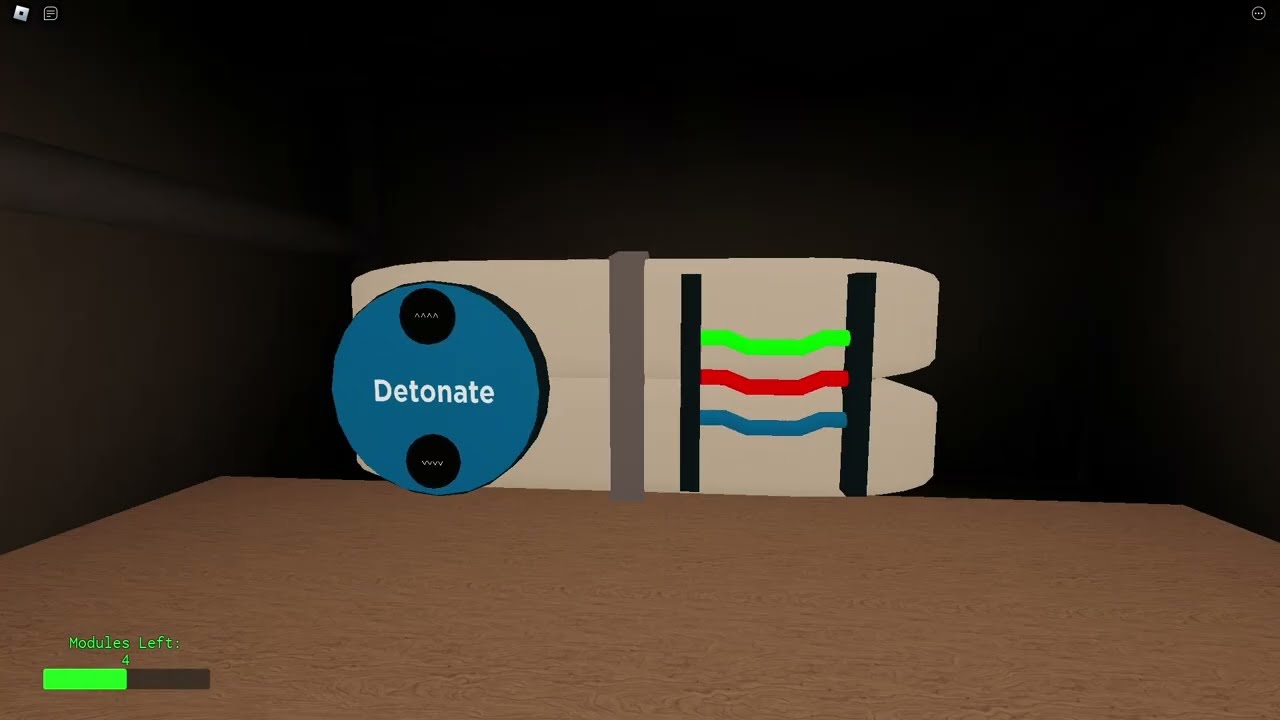The image appears to be a simple, computer-generated scene that resembles an interface or screen from a video game, possibly created using a basic paint program. The background is predominantly black, emphasizing the foreground elements. At the bottom of the image, there is a brown surface that could either represent a wooden table or floor. 

In the lower left corner, there is a progress bar that says "Modules Left" with the number 4 next to it. The progress bar is half-filled with a bright lime green color. 

Central to the image is a depiction of what seems to be a bomb. On the left side of the bomb is a prominent dark blue circle with the word "detonate" written in white. Above the circle are two black dots that may resemble buttons. 

To the right of the blue circle, there are two vertical black lines connected by horizontal wires. These wires are colored green, red, and blue, making them stand out against the black background, resembling a ladder or wires to be cut. 

The overall impression is that of a bomb-defusing interface, presented in a simplistic and somewhat amateurish graphical style.